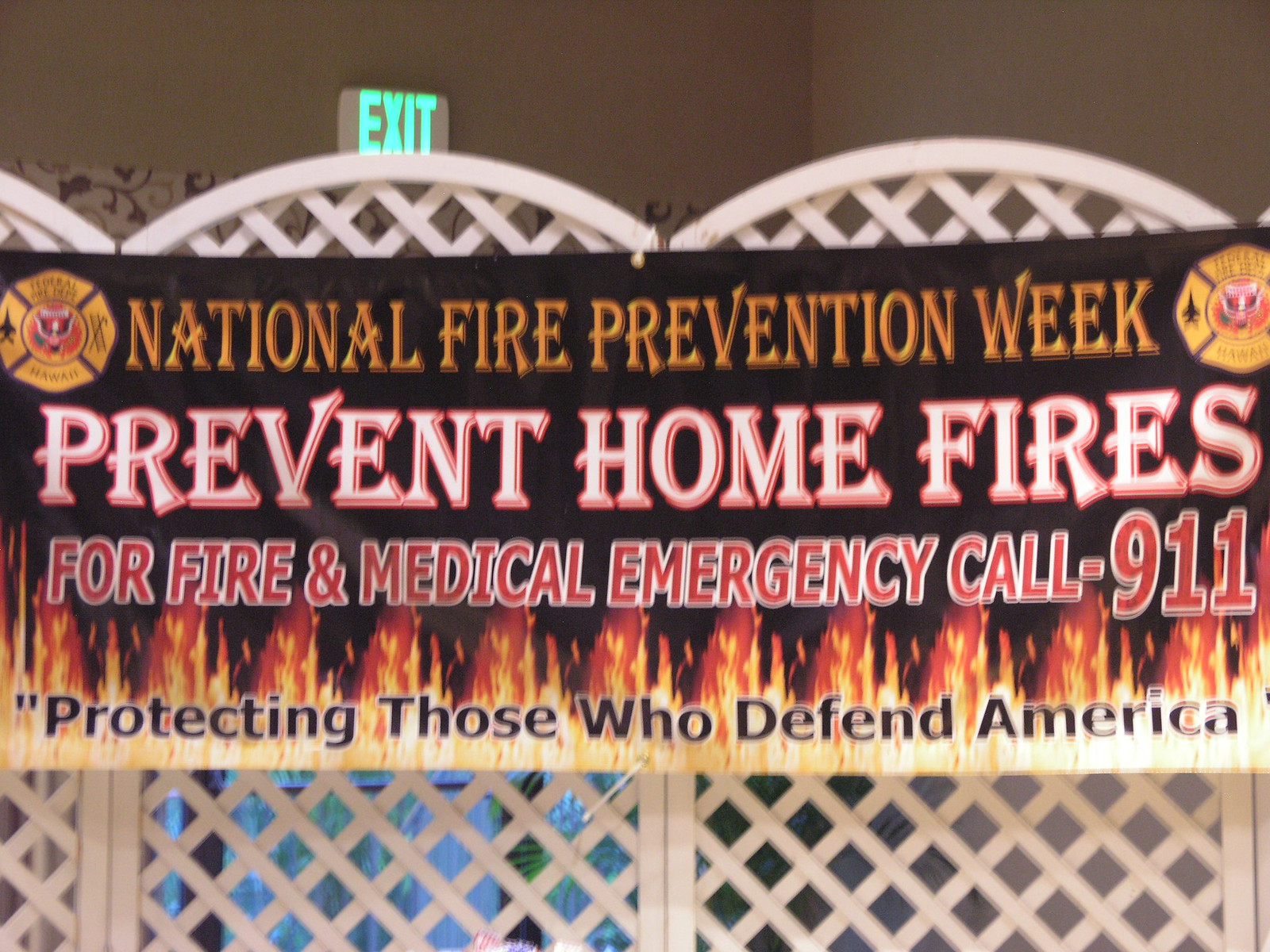In this image, there is a white, lattice-style fence composed of three sections, which appears behind a prominently featured banner. At the top of the image, a green exit sign with white lettering is visible against the white wall. The banner itself is black and includes several detailed components. At the very top of the banner, there are two gold-trimmed fire department symbols with red centers. The banner's main text is in bold yellow, reading "National Fire Prevention Week" in large, striking letters. Below that, in large white font with red borders, it says, "Prevent Home Fires." Further down, in red text with a white border, the banner directs, "For Fire and Medical Emergency Call 911." At the very bottom of the banner are orange and red flames, and below this, in black text with a white outline, it states, "Protecting those who defend America." The entire scene appears to be a mix of indoor and outdoor elements, possibly in an event space, illuminated by the overhead exit sign.